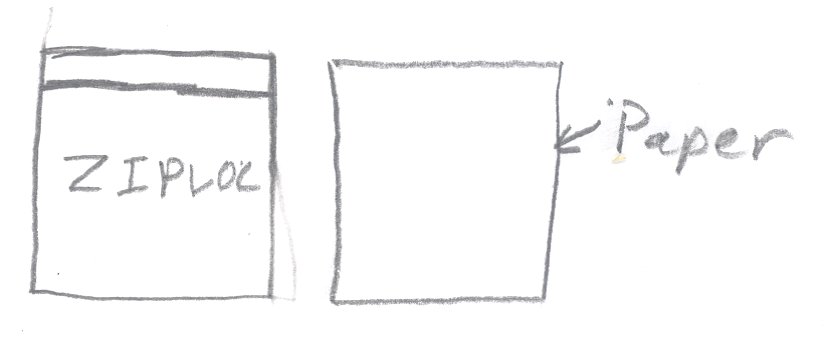The image features a rudimentary drawing on a plain white background, likely done with a broad-tipped pencil, possibly a carpenter's pencil. On the left side of the drawing, a square is depicted with its top line having been traced several times, resulting in a darker, more pronounced appearance compared to the side and bottom lines. Just below this top line, there is a small white gap, followed by another horizontal line that has also been repeatedly traced to enhance its darkness. Within this square, the word "ZIPLOC" is inscribed in capital letters, albeit sloppily, with uneven alignment and incomplete form – the final 'C' appears more like an 'L'.

Adjacent to this square is another, similarly sized square. Unlike the first, this one features uniform line thickness and darkness across all four sides. An arrow points down and to the left, touching the right side of this second square. Next to the arrow is the word "PAPER" written with a capital 'P' followed by lowercase letters. There appears to be a stray dot near the 'P', likely an accidental mark.